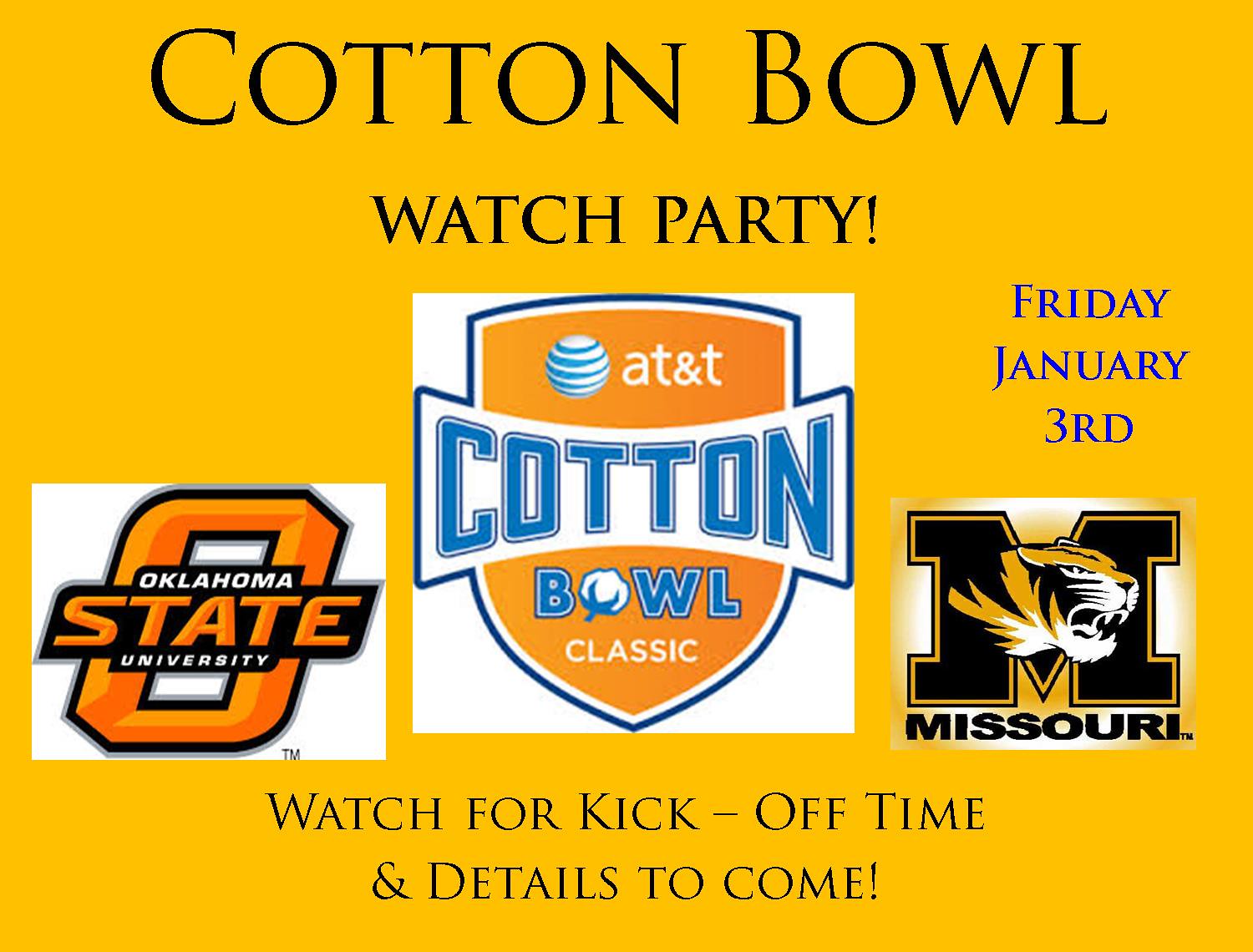The image is a computer-generated advertisement for a Cotton Bowl watch party set against a vibrant yellow background. At the very top, bold black text announces "Cotton Bowl Watch Party" with "Friday, January 3rd" in blue text to the right. Central to the image is the Cotton Bowl emblem, a prominent gold shield featuring the AT&T logo at the top and a white circle with blue lines representing a football. In blue text, "Cotton Bowl Classic" is inscribed on the shield. Flanking the emblem, to the left, is the Oklahoma State University logo—a large orange "O" with "Oklahoma State" written across it. To the right is the Missouri Tigers logo, characterized by a massive black "M" with a black and yellow tiger's head. At the bottom, black text advises viewers to "watch for kickoff time and details to come."